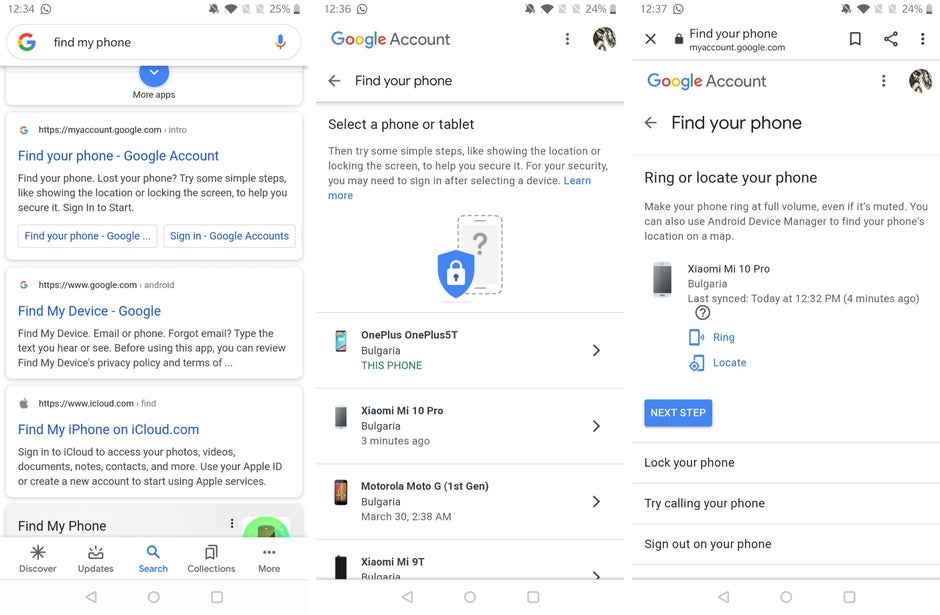A series of three smartphone screen captures illustrate the steps to locate a lost device. 

In the first image, someone has typed the query "find my phone" into the Google search bar, yielding a list of results. They appear to have selected an option titled "Find your phone - Google Account."

The second image shows Google's "Find your phone" page, asking the user to select a device from a list of their connected devices. The chosen device, a Xiaomi Mi 10 Pro, shows up on the list and is indicated to be in Bulgaria.

The third image provides options for the user to either ring or locate their phone, completing the process to help them recover their lost Xiaomi Mi 10 Pro.